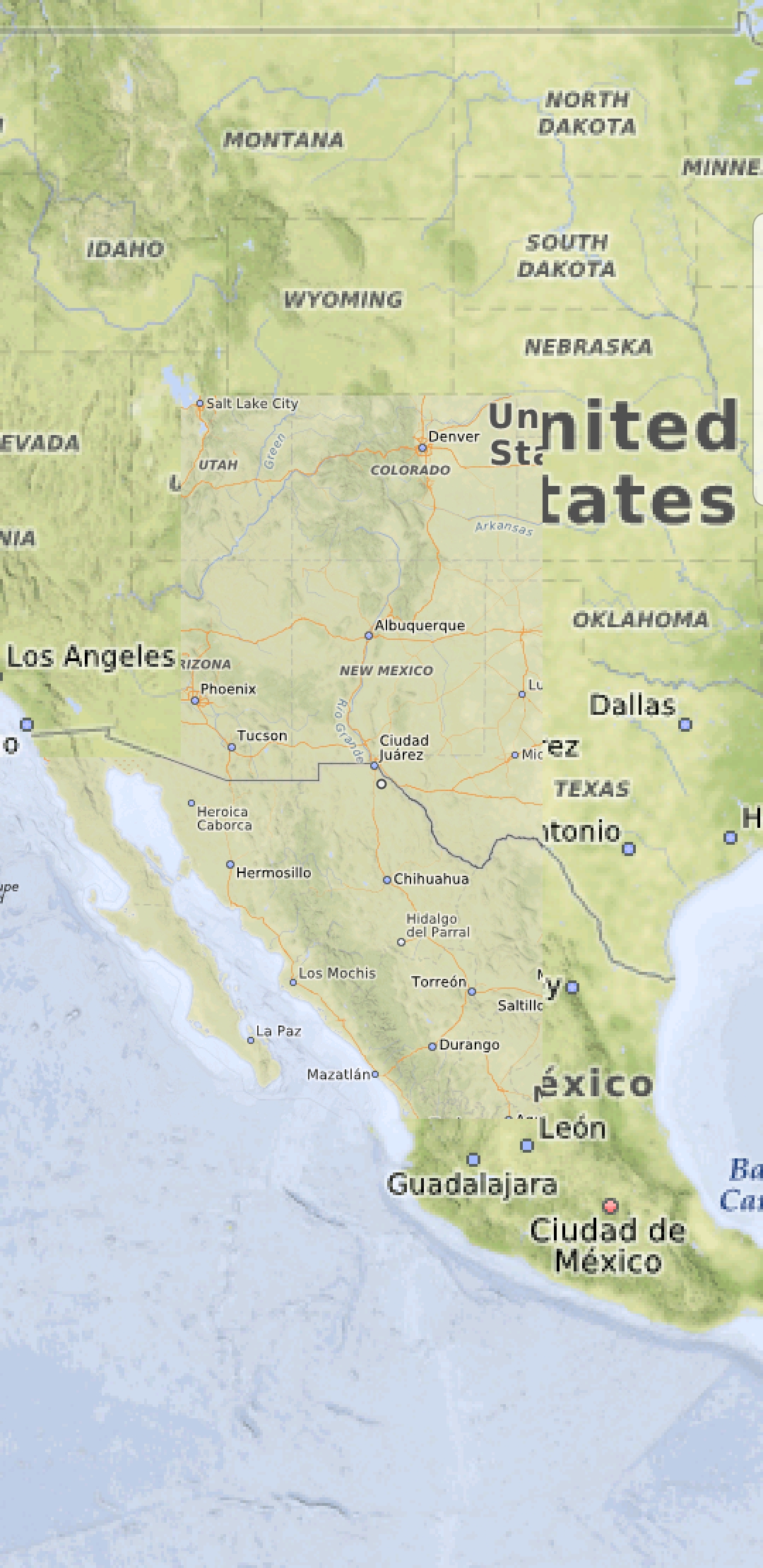The image portrays a visually intriguing map segment of the United States and Mexico, combining elements of both painted and drawn styles, suggesting a layered composition. A notable feature is the overlap of two maps: an outer map predominantly in pale green hues showcasing state names and major cities, and an inner map in a lighter green or tan hue with finer details, displaying more cities and routes. 

The text on the map is partially cropped, with "UNITED STATES" being truncated, showing only pieces like "UN" followed by "NITED" and "S-T" with part of "A" then "T-A-T-E-S". Prominent among the details are cities such as Dallas, indicated by a silver dot bordered in black, and other cities like Albuquerque, Phoenix, Tucson, Salt Lake City, and Denver on the inner map, alongside Ciudad Juarez and Chihuahua in Mexico.

The map employs a pastel light blue to depict water bodies, with traces of medium blue, while land areas transition across shades of pale to dark green, indicating varied landscapes. Red-orange lines highlight routes across the map. States such as Texas are distinctly italicized, bolded, and shadowed in white. Towards the left, 'Los Angeles' is visible, and above it, a partially cropped "N-I-A" likely representing California, with "Nevada" shown without its initial 'N'. This combination and superimposition of maps create a rich, multilayered depiction of the region.